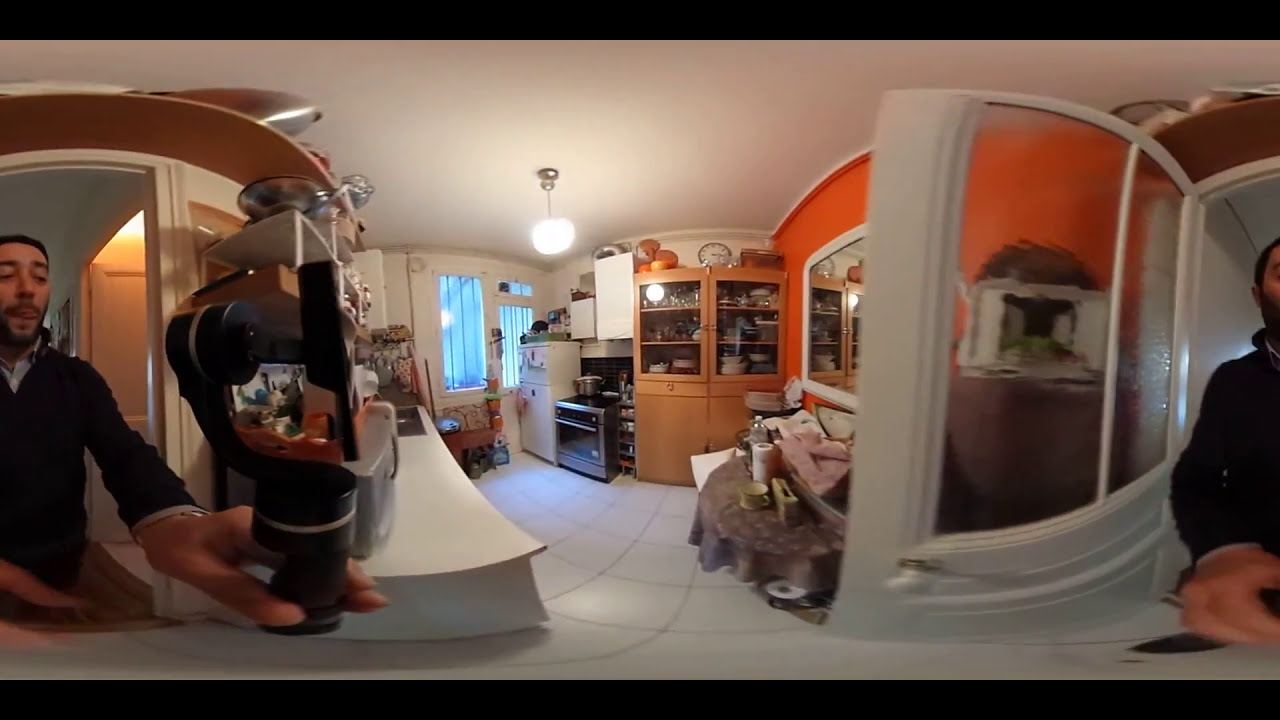In this panoramic indoor shot, we see a man with dark hair, a beard, and a mustache wearing a dark-colored sweater standing on the left side and partially on the right due to the image's wrap-around effect. He holds a tool or possibly a coffee cup and seems to gaze towards, but not directly at, the camera. The room appears to be a kitchen, with white tile flooring, a white refrigerator, a black stove, and white countertops. High open shelves, likely holding pots, pans, or bowls, and a wooden cupboard with glass-topped doors containing dishes are visible. Above the cupboard, there is a clock and some stacked baskets. The walls are predominantly white with a notable bright orange section featuring a large mirror. A table cluttered with various items sits against this orange wall. Windows with blinds allow natural light in, suggesting the photo was taken during the day. A white ceiling light hangs centrally, illuminating the room. The overall composition includes a blend of colors, including white, orange, yellow, black, gray, tan, blue, and pink.